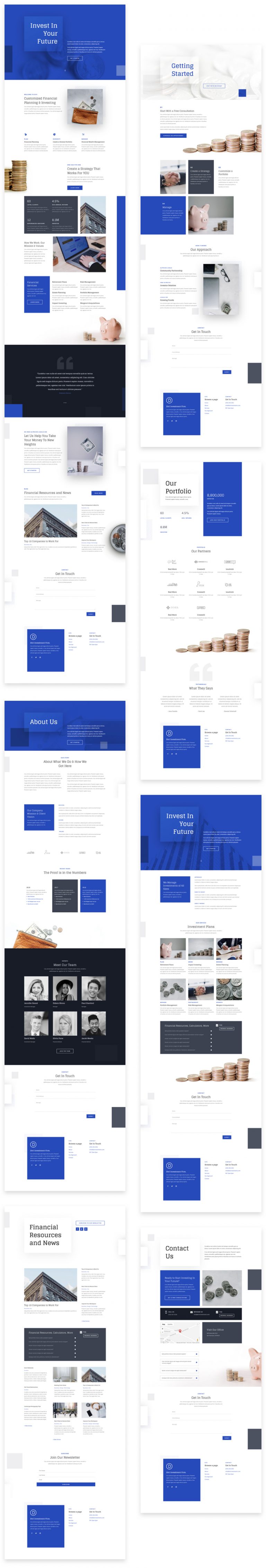The image comprises several screenshots, approximately 8 to 10, from a financial information website, each depicting different sections of the site. The first screenshot highlights an "Invest in Your Future" page, which appears to set the stage for prospective investors. Following this, the "Getting Started" page provides an introductory guide for new users. Another page laid out in a blog-style format lists various articles, offering insightful reads and updates. The "Our Portfolio and Our Partners" page showcases the company’s investment portfolio and includes testimonials from collaborators. Moving on, the "About Us" page details the company’s mission, history, and values. The "Meet Our Team" section introduces key team members, while also featuring a "Get in Touch" section for inquiries. Another screenshot reiterates the "Invest in Your Future" theme but delves deeper into specific investment plans. The "Financial Resources and News" page is text-heavy, containing the latest financial news and resources. Finally, the "Contact Us" page provides multiple avenues for communication, reinforcing the "Get in Touch" section to facilitate user interaction.